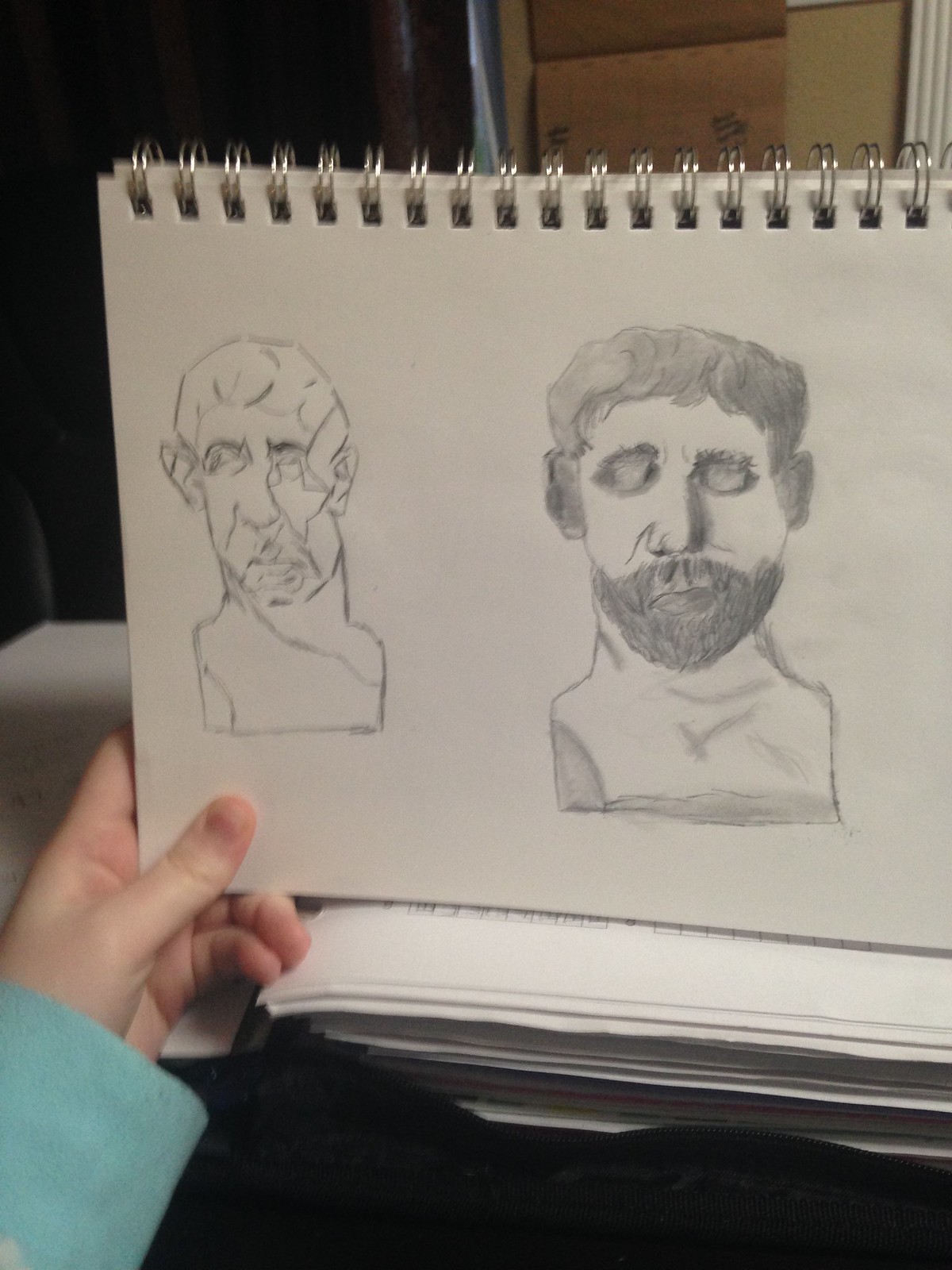This digital photograph, taken indoors, captures a person's left hand, clad in a blue sleeve, holding up a sketchbook with a wire ring binder. The background is predominantly black on the upper left, transitioning to what appears to be a couch or chair. A tan cardboard box adorned with Asian script sits to the right, adjacent to a light tan corkboard. Below this arrangement, a white piece of mortar edging is visible.

In the foreground, a black fleece with a visible zipper extends across the bottom, partially covering a substantial stack of white papers. The sketchbook, held in a light-skinned hand, features two pencil-drawn busts of men. The drawing on the left is a simplistic, rough sketch of a man's face, resembling a stone statue. The drawing on the right is more detailed, with shaded hair, dark circles around the eyes, and a full, meticulously shaded beard and mustache. This photograph meticulously captures the intricate details and contrasts of the surrounding objects and the artistic renditions within the sketchbook.